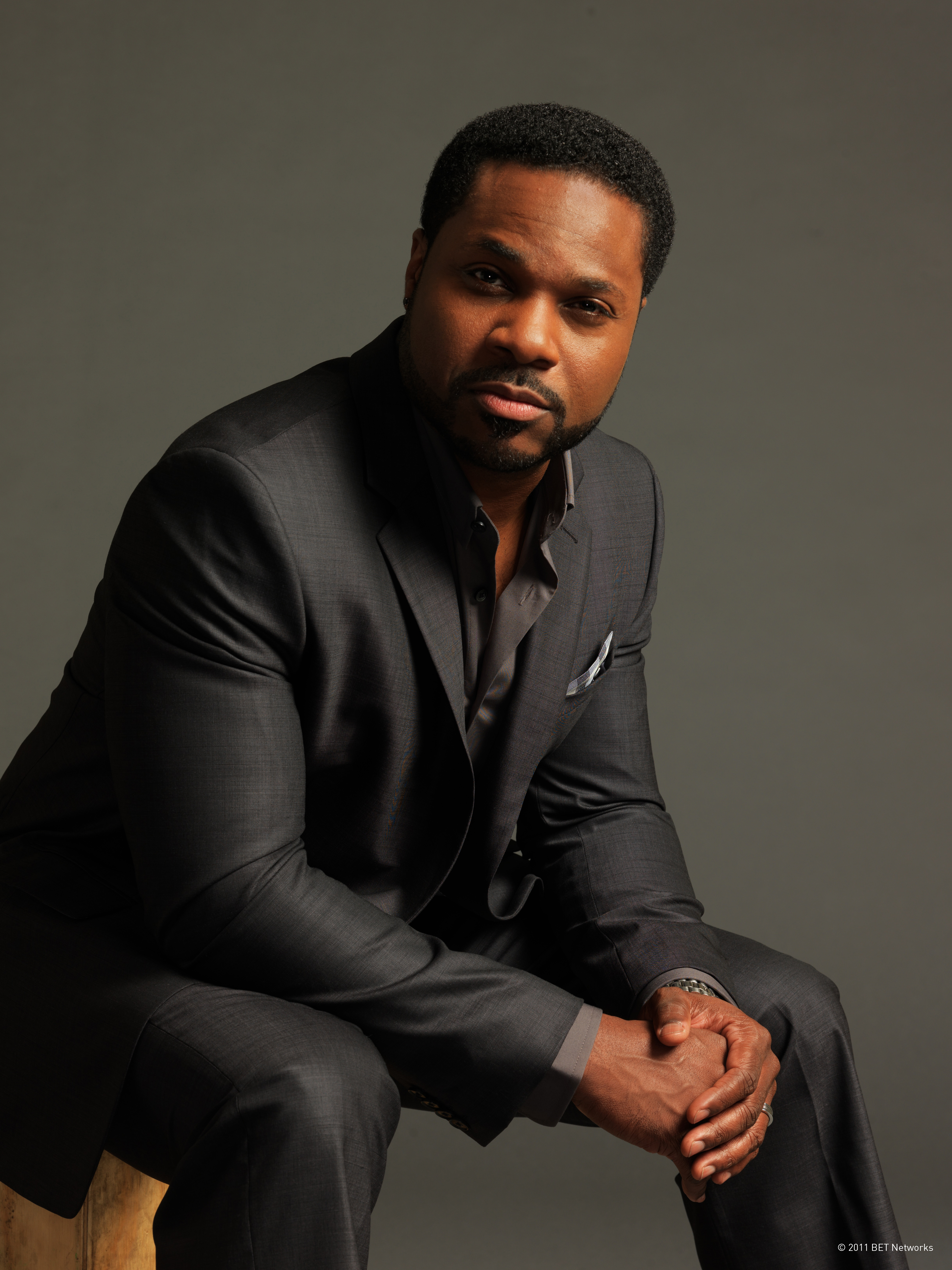The studio photo features a middle-aged black man sitting on a wooden bench against a grey background. He's wearing an open, all-black suit paired with a black shirt. Accessories include a silver ring and a silver watch, adding an elegant touch to his look. The man sports a stylized beard and a short afro, with his skin tone lit predominantly from the left side, suggesting careful studio lighting. He gazes directly into the camera with a serious expression, his right eyebrow raised. This pose, coupled with his attire, lends a composed and sophisticated aura to the image. In the lower right corner, the credits for BET Networks are visible, indicating that this is likely a promotional photograph for the network. Some might find a resemblance to Malcolm-Jamal Warner, known for his role in "The Cosby Show."